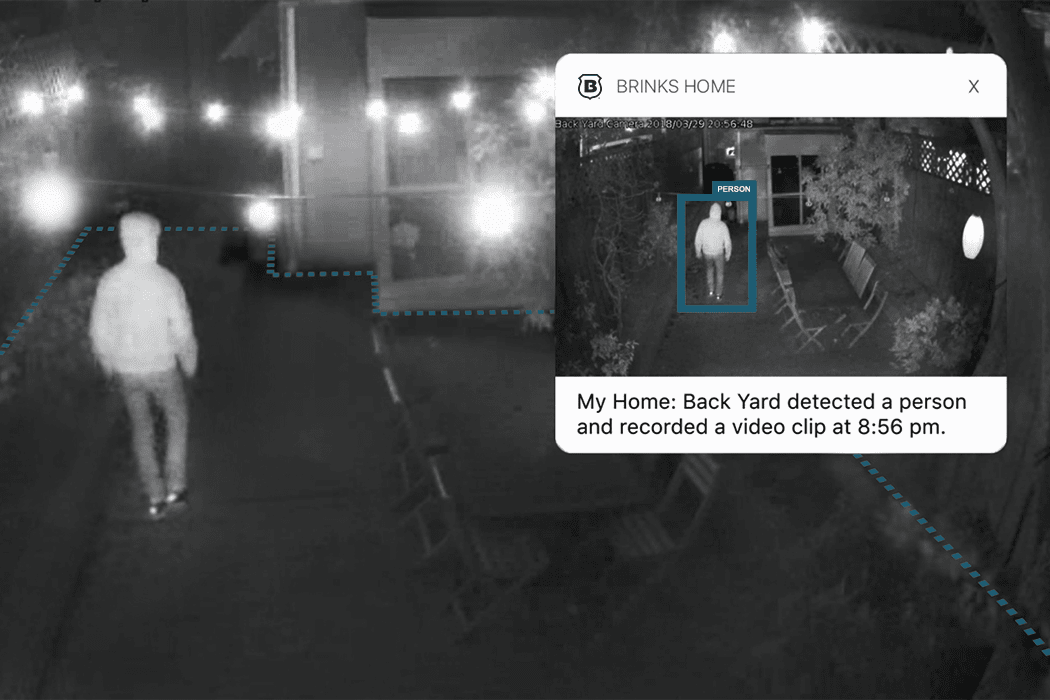The image appears to be a screenshot of a nighttime security camera feed from a home surveillance system, identified by the Brinks Home logo and accompanying informational text. The main photo, taking up the majority of the space, provides a detailed view of a backyard setting. On the right side of the image, there's a patio area with a table and chairs, bordered by shrubbery and a wooden, slatted lattice fence. Twinkling string lights are strung overhead, casting a decorative glow over the scene. A prominent blue, dashed line outlines the perimeter of the patio, near the ground.

To the left of the table, an individual clad in a light-colored hooded jacket, pants with a grey stripe, and sneakers is captured mid-step, walking away from the camera. This individual's presence is highlighted by a turquoise blue rectangle. Additional shrubbery is visible to the left of the person. In the background, you can see part of the house, including a back glass door with a tree partially overhanging it, and a light post.

Inset into the top right corner of the main image is a smaller photo with a Brinks Home caption that reads, "My Home Backyard Detected a Person and Recorded a Video Clip at 8:56 PM," confirming the time and nature of the activity.